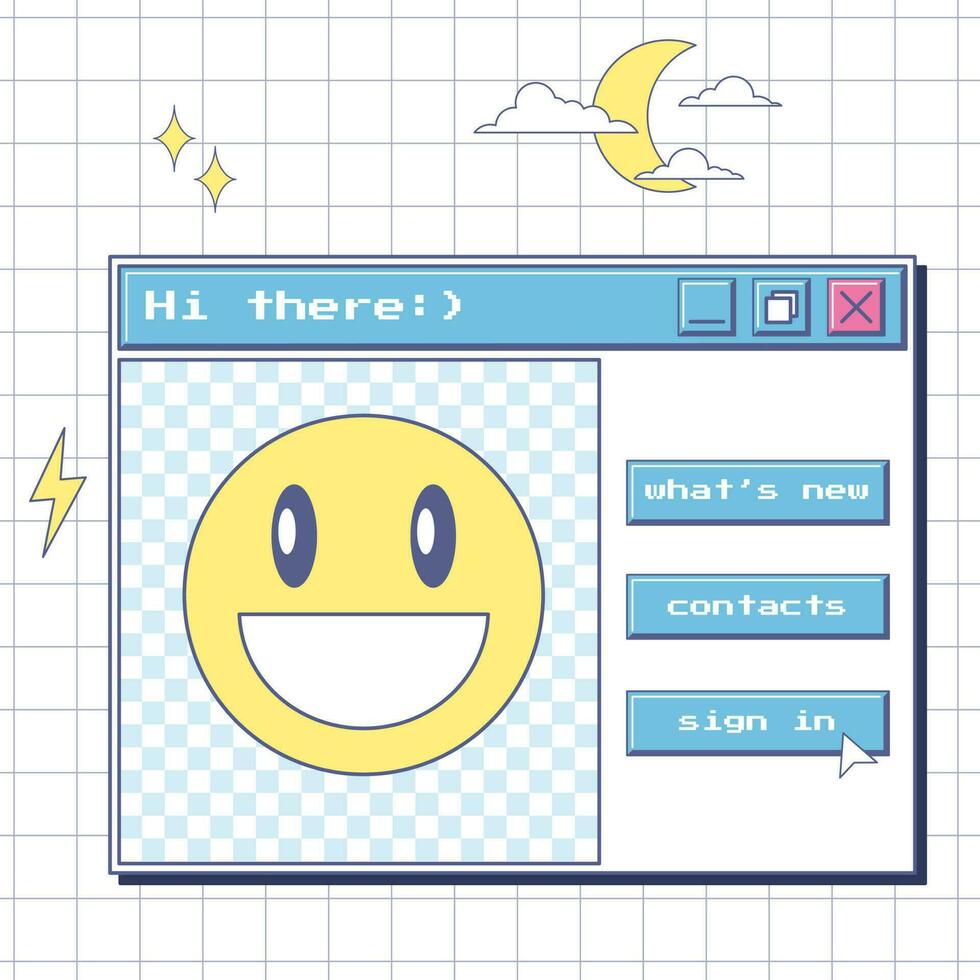The image features a white background with a grid pattern of black, gray squares, resembling graph paper. Scattered across this backdrop are various pixelized clipart graphics: a yellow moon surrounded by white clouds, two yellow diamond stars, and a yellow lightning bolt. Central to the image is a computer pop-up box with a distinctly retro feel, reminiscent of an old-fashioned Windows chat room or AIM AOL instant messenger. The box displays the greeting "Hi there" and includes the options "what's new," "contacts," and "sign in," with a computer mouse icon hovering over the sign-in option. In the top-right corner of the pop-up are the classic minimize, maximize, and close buttons, with the close button being red. To the left of the text is a large, cheerful smiley face with baby blue and white checkered squares behind it, radiating a sense of nostalgia. The overall color scheme includes shades of yellow, pale yellow, black, white, and baby blue, enhancing its retro computer graphic vibe.